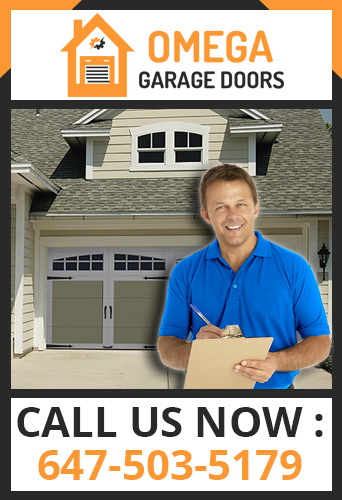This image showcases a house with beige siding, featuring a two-door garage. In front of the house stands a man dressed in a blue collared polo shirt, holding a clipboard and pen. The advertisement prominently displays the logo for Omega Garage Doors, with "Omega" in orange and "Garage Doors" in black. An additional graphic element includes an orange house encapsulated within a yellow-orange and black circle. The text "Call us now" is printed in black and orange, followed by the contact number (647) 503-5179.